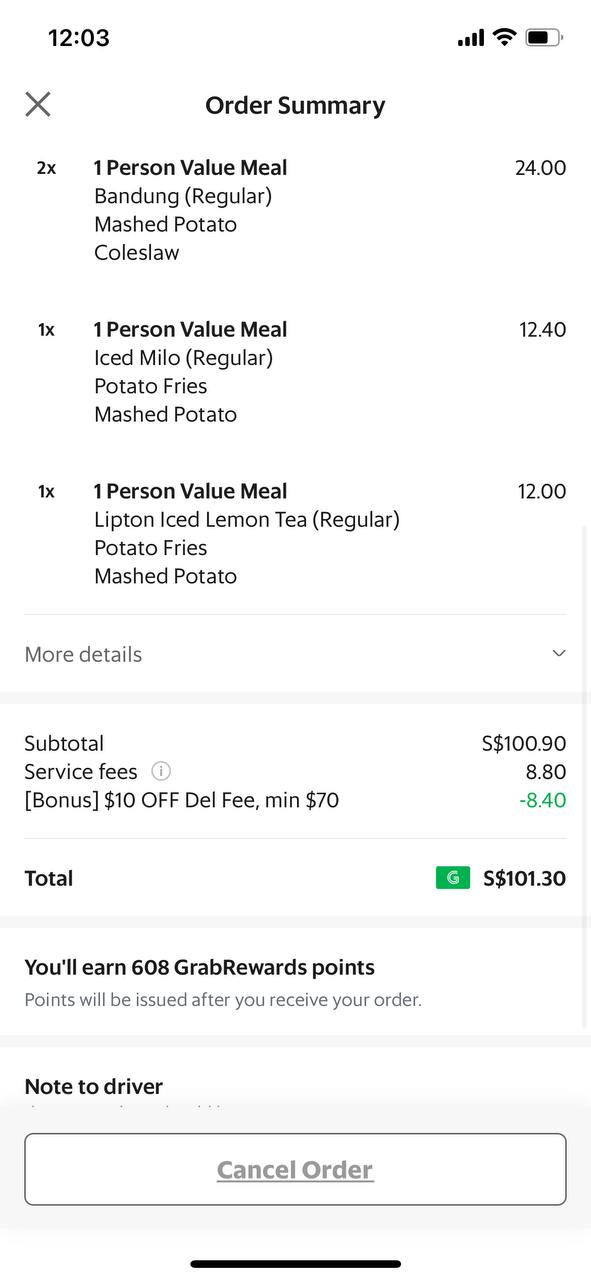A screenshot capturing an order summary for a food delivery, displaying various interface elements and details of ordered items. The timestamp "12:03" is prominent at the top in black text on a white background. Icons indicating full data service (4/4), full Wi-Fi signal (3/3), and approximately three-quarters battery life are displayed alongside.

The screen features a grey 'X' button to close the window, and the heading "Order Summary" in bold black text. The order includes:

- **Two 1-Person Value Meals**: Bandung Regular, mashed potato, and coleslaw for a total of $24.00.
- **One 1-Person Value Meal**: Iced Milo Regular, potato fries, and mashed potato for $12.40.
- **One 1-Person Value Meal**: Whipped and Iced Tea Regular, potato fries, and mashed potato for $12.00.

Additional order details show a subtotal of $100.90, service fees amounting to $8.80, and a $10 bonus off. A delivery fee adjustment shows a credit of -$8.40 due to the minimum order requirement, culminating in a total of $101.30. The customer will earn 608 Crab Reward points, which will be issued once the order is received.

At the bottom of the screen, there is a white "Cancel Order" button, and a black line suggesting the option to swipe up to view more content on the device.